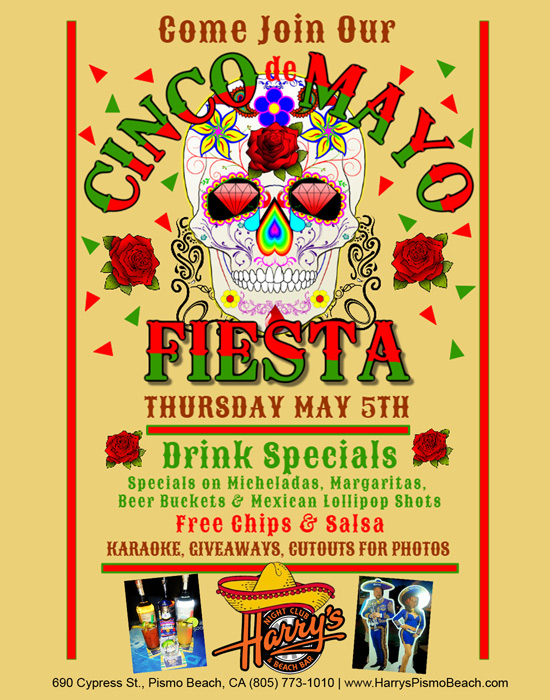This vibrant, beige-background poster advertises the "Cinco de Mayo Fiesta" event, hosted by Harry's Nightclub and Beach Bar at 690 Cypress Street, Pismo Beach, California. The festivities occur on Thursday, May 5th, as prominently displayed in brown text. At the top, the poster invites everyone to "Come Join Our" in brown lettering, followed by an arched "Cinco de Mayo" in alternating red and green letters, overlaid on a sugar skull with diamond eyes and a rainbow, upside-down heart for a nose. Surrounding the skull are intricate black filigree patterns flanked by red roses, amid a scattering of red and green triangle confetti. Below the skull, the event is denoted as "Fiesta" in matching green and red text, partially overlapping the skull's chin.

An enticing array of drink specials is listed in green text, featuring Micheladas, Margaritas, Beer Buckets, and Mexican Lollipop Shots, bordered by roses. Further promotions include "Free Chips and Salsa" in red text, and additional highlights like karaoke, giveaways, and photo cutouts, mentioned in brown. The bottom part of the poster showcases images of liquor bottles and cocktail glasses, enhancing the festive spirit. Centrally placed is Harry's logo with a sombrero on top, asserting its beach bar identity.

Finally, below the images, the poster provides essential venue information in small black print, including the full address and contact number (805-773-1010), with the website "www.harryspismobeach.com" detailed at the very bottom. Accompanying these details are images of people dressed in traditional blue mariachi outfits, highlighting the cultural flair of the event.